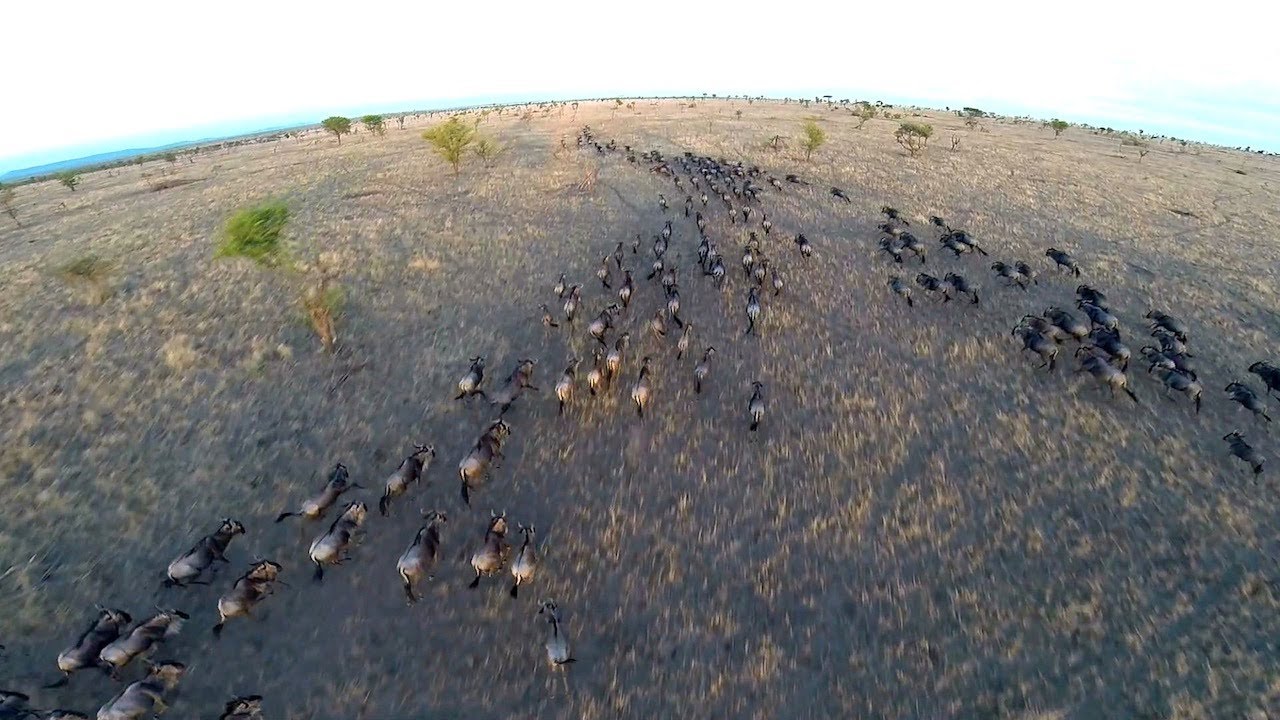A panoramic image captures the vast plains of the African savanna, teeming with hundreds of wildebeests in a breathtaking display of migration. The terrain, a mixture of muddy, moist grasslands and patches of brown grasses, stretches endlessly under a hazy white sky, marked only by narrow bands of blue near the horizon. The fisheye lens accentuates the expanse, curving the landscape into a broad, sweeping vista. Scattered trees punctuate the plain, more densely situated towards the right. From opposite sides of the panorama, two distinct lines of wildebeests converge into a Y-shaped formation, merging into a single, unified mass as they race away into the distance, creating a mesmerizing spectacle of nature's grandeur.